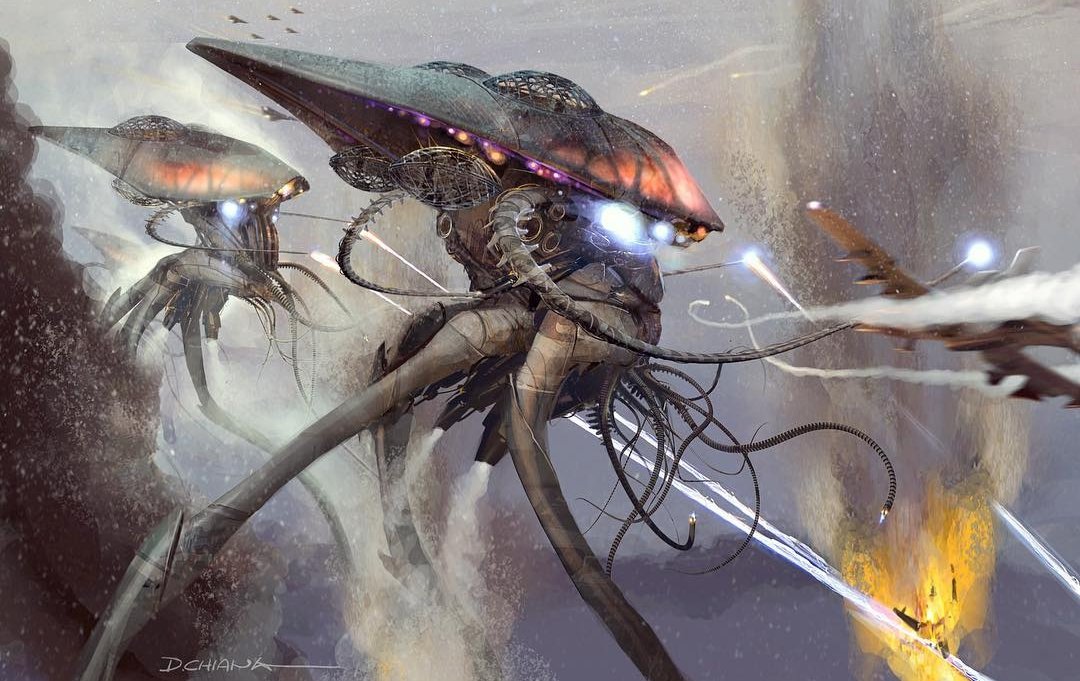The image depicts a highly dynamic, action-packed fantasy battle scene featuring two massive, futuristic mechanical creatures engaged in combat with various airplanes. These towering machines resemble a hybrid of airplanes and walking entities, standing so tall on their spindly legs that they engage in aerial dogfights. The mechanical beings possess heads that project backward, adorned with lights on their undersides, and wield multiple tentacle-like arms. One creature appears to be launching lasers or rockets from two of its appendages, while the other is grasping a fighter plane.

The battlefield is chaotic with numerous explosions, especially noticeable in the lower right corner where a plane has been downed, surrounded by a burst of yellow flames and flying debris. Missiles streak through the sky, and a mix of old-fashioned and modern fighter jets — some from the 1950s and others more contemporary — are engaged in the fray, particularly in the upper left corner where they seem to be offering support. The backdrop of the image is gray and obscure, adding to the intensity of the scene. On the bottom left, the name of the presumed artist, 'D. Chiana' is inscribed, lending a personal touch to the vibrant and chaotic tableau.